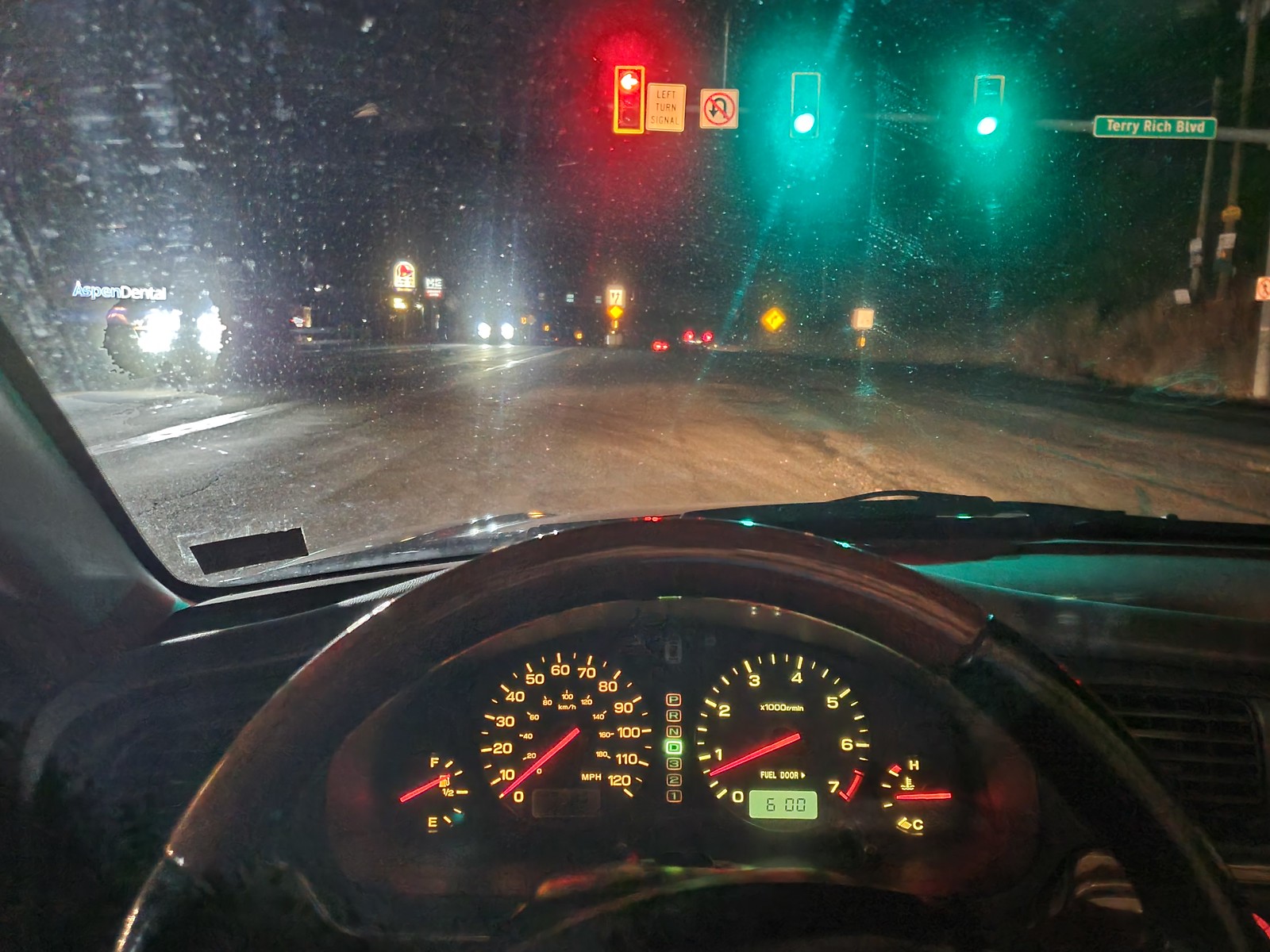The photograph captures the interior view of a car's dashboard at nighttime. The dashboard is illuminated by the vehicle’s lights, with the speedometer showing a current speed of approximately five miles per hour. To the left of the speedometer, other typical car dials are visible. The steering wheel is seen in the foreground, its color appearing to be either black or gray, difficult to discern due to the low lighting. The dashboard also features labels such as "Fuel Door" and the number "6".

Outside the car, the windshield, which appears slightly dirty, reveals a city street scene brightly lit by numerous street lights. A Terry Rich Boulevard street sign is clearly readable. The traffic light ahead shows a red left turn arrow and two green lights for going straight. The headlights of other vehicles shine through the windshield. Off to the left in the distance, the illuminated sign for "Aspen Dental" is distinguishable, adding context to the location.